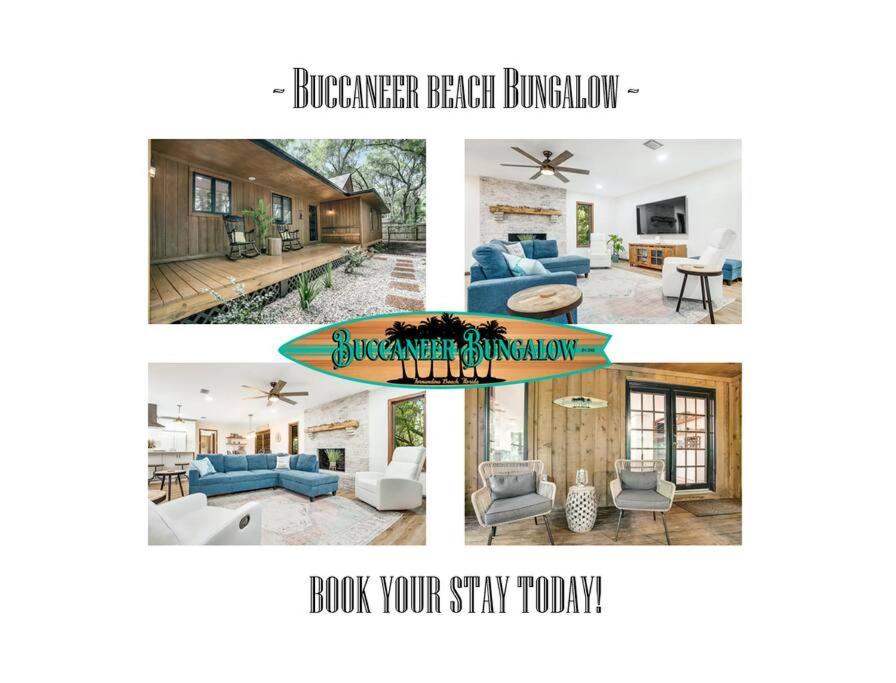The advertisement features a composite of four photographs showcasing the Buccaneer Beach Bungalow, with the text "Buccaneer Beach Bungalow" prominently displayed at the top. Central in the layout is a design that connects all four images, bordered in green with a wood center adorned with tree silhouettes, reading "Buccaneer Bungalow" in aqua blue, and the phrase “Book your stay today” at the bottom.

The top left photograph captures the rustic exterior of a bungalow made from unpainted wood, fronted by a gravel walkway. Two rocking chairs sit on the covered porch, separated by a plant. The top right image offers a glimpse into the cozy living room featuring hardwood floors and an aqua-colored sofa paired with blue pillows. A fireplace with a mantle, a wooden TV stand below a large flat-screen TV, a white recliner next to a round end table, and a ceiling fan complete the room’s welcoming ambiance.

The bottom left photograph presents a different angle of the living room, emphasizing the aqua sofa and providing a clearer view of the fireplace. Lastly, the bottom right image showcases another deck or porch, with two distinct types of chairs facing a wooden facade. Behind the chairs are large sliding glass doors, leading into the well-lit interior that may include a bar or kitchen area, with visible furnishings like armchairs and a floor-to-ceiling window comprised of multiple panes.